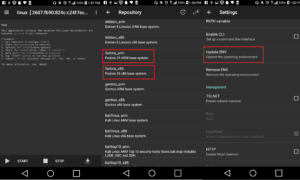This image comprises three side-by-side screenshots, each of notably low resolution, making the text difficult to read. The status bar across all three screenshots displays several icons including the airplane mode icon, a network signal bar, a headphone connection icon, and a Wi-Fi signal icon. The first screenshot is unclear in its contents, while the second and third screenshots are more identifiable. At the top of the second screenshot, the word "Repository" is visible, and this image features two details marked in red. The third screenshot is labeled "Settings" at the top and has one detail highlighted in red. The color scheme across these screenshots includes black, red, grey, and white tones.